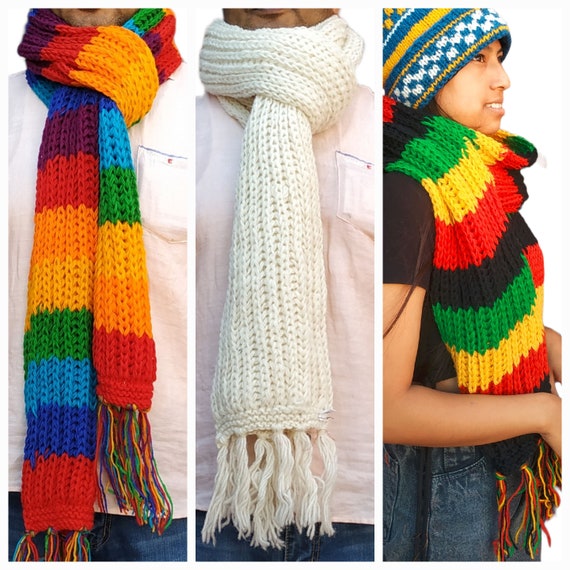The image showcases three separate portrait photographs of people wearing scarves, each with its distinctive style and colors. The first photo features an individual wearing a multi-colored scarf with an intricate pattern of red, blue, lighter blue, green, orange, darker orange, and red mixed with black stripes, all knotted neatly around their neck. The person is dressed in a white shirt and jeans, though their face is not visible. The second photo depicts what appears to be the same person, now wearing a simple, elegant white knitted scarf, draped gracefully over a pale pink shirt and blue jeans, again without the person's face shown. The third photo captures a different individual, an Asian woman seen from a side profile, smiling warmly while wearing a blue, yellow, and white hat. Her multi-colored scarf, displaying alternating stripes of green, yellow, red, and black, complements her black short sleeve t-shirt and jeans. Each scarf features decorative strands hanging from the bottom, enhancing their textured, cozy appearance.